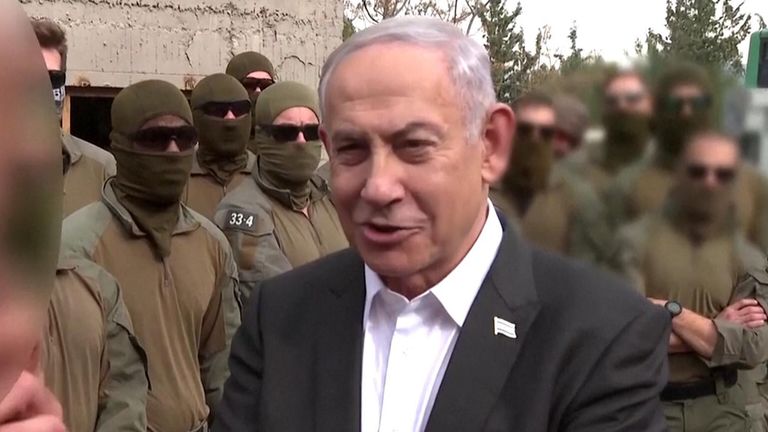The image depicts an older gentleman, likely a politician, with grayish-white hair combed to the side and cut short. He is wearing a black suit jacket over a white collared shirt, adorned with an American flag pin on the right lapel. His lips are slightly parted, suggesting he may be speaking. The man has a slight smirk on his face and appears to be in a greeting posture. Surrounding him are men dressed in dark green and olive green military-style uniforms. These individuals are wearing balaclavas and dark sunglasses, masking all but the tops of their foreheads and bridges of their noses. To the left of the politician, one man is clearly visible, bearing a patch on his shoulder with the number "334" in white text, while others in the background are blurred or out of focus. The collective image implies a connection or interaction between the politician and the masked men.